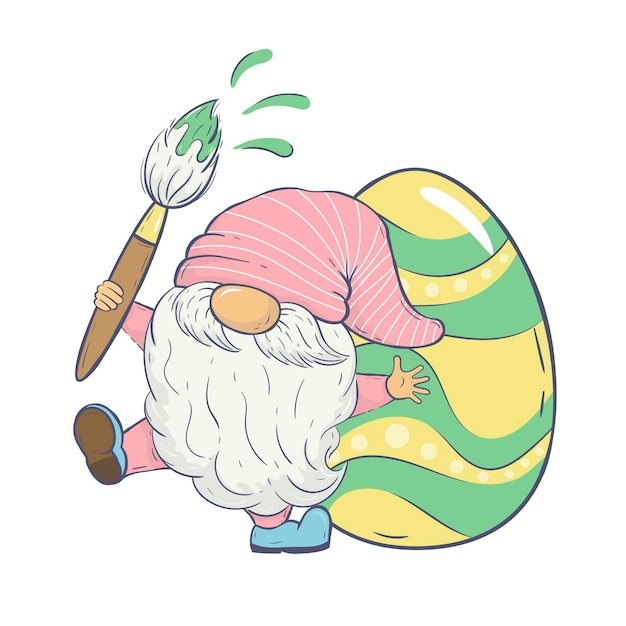This colorful illustration features a friendly, humorous, gnome-like character with a flowing white beard and mustache. His large, round, beige nose protrudes from beneath a pink nightcap adorned with white stripes that drapes over his eyes. Emerging from his beard are two stubby pink legs and blue shoes with tall rounded toes. He holds a paintbrush in his right hand, characterized by a wooden handle and a gold clasp, with its white bristles covered in lime green paint that splashes outward.

Behind the character, and positioned towards the right, stands a large, vertically-oriented Easter egg. The egg, which is larger than the character himself, has a yellow background accentuated by wavy olive green stripes. These stripes include sections with white polka dots and a highlighted reflection in the top right. The background of the entire scene is completely white, emphasizing the vibrant details and cheerful demeanor of the character.